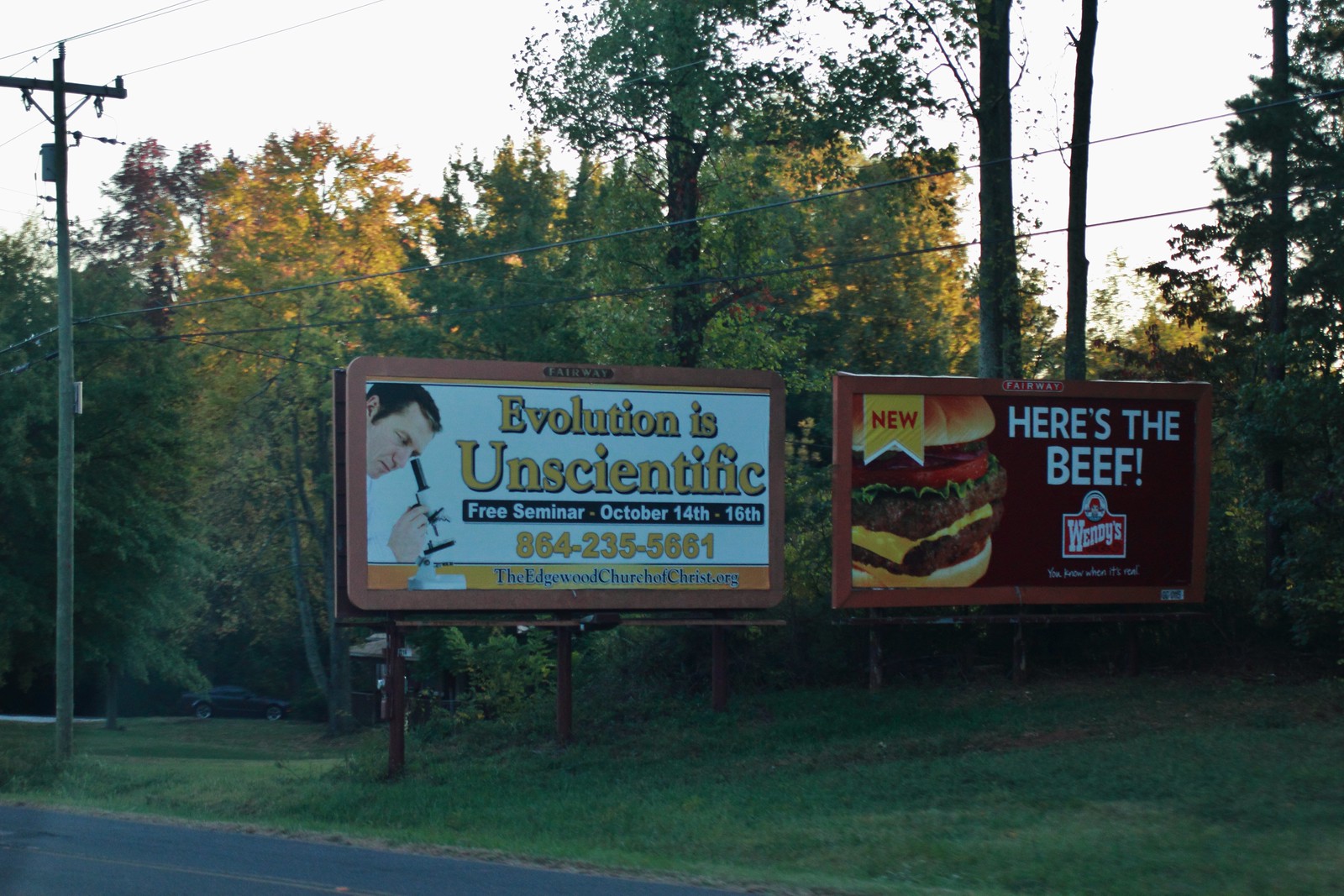This outdoor photo, captured during late afternoon as indicated by the long shadows on the green and golden-hued trees, features a pair of detailed billboards along a roadside lined with power poles. The right billboard promotes Wendy's with a bold statement, "Here's the Beef," showcasing an appetizing double meat burger beneath a "New" banner, and the Wendy's logo accompanied by the word "Fairway" at the top. The left billboard, with a gold and white color theme, declares, "Evolution is Unscientific," and depicts a man peering through a microscope. This sign also advertises a free seminar from October 14th to 16th, providing contact information including a phone number and a website, edgedwoodchurchofchrist.org.